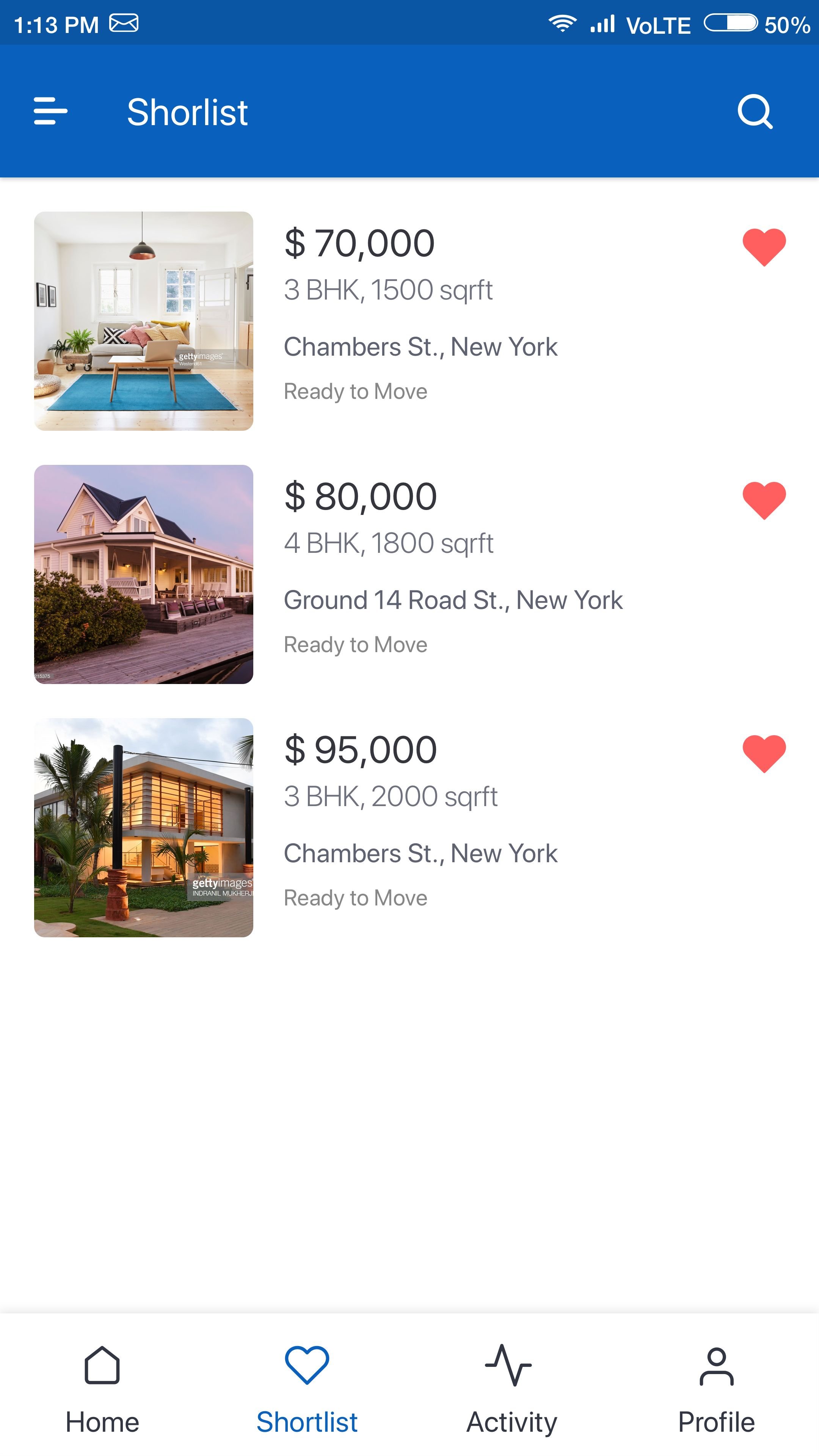This screenshot, taken from a mobile phone, clearly displays the device's status bar at the top, indicating a time of 1:13 p.m., an envelope icon, a Wi-Fi signal bar, the provider name "Volte," and a battery level of 50%. The content on the screen appears to be from an Airbnb or real estate app featuring several property listings. The first listing shows a price of $70,000 for a 3BHK apartment with 1,500 square feet located on Chambers Street, New York, accompanied by a photo of the property and a heart icon for favoriting the listing. Other listings follow, with one priced at $80,000 on Ground 14th Road Street and another at $95,000. At the bottom of the screen, options for profile, activity, and shortlist are visible.